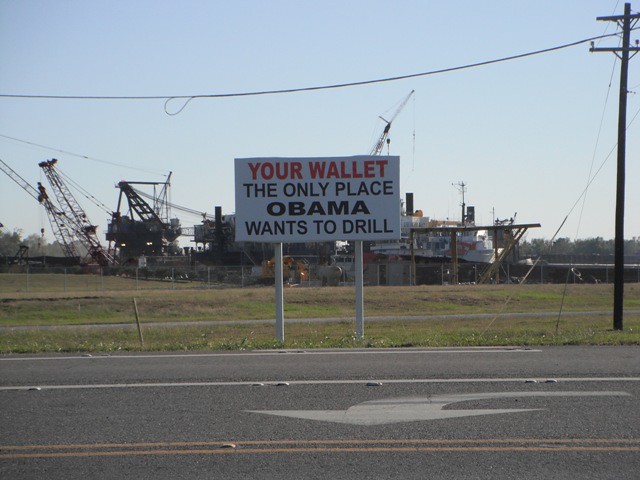This photograph, taken from or near the roadside, captures a provocative sign mounted on two wooden posts. The sizable rectangular sign features a bold and colorful message. In large red capital letters, the top of the sign reads, "YOUR WALLET," with the subsequent line proclaiming in black capital letters, "THE ONLY PLACE OBAMA WANTS TO DRILL." The name "Obama" is emphasized in bold lettering. Behind the sign, an oil rig is visible, clearly intended to reinforce the political statement made by the sign. The scene is bathed in daylight, under a clear blue sky without a single cloud in sight. Power lines are also visible, stretching across the background. The image evokes a politically charged sentiment against former President Obama concerning energy policies and economic matters.